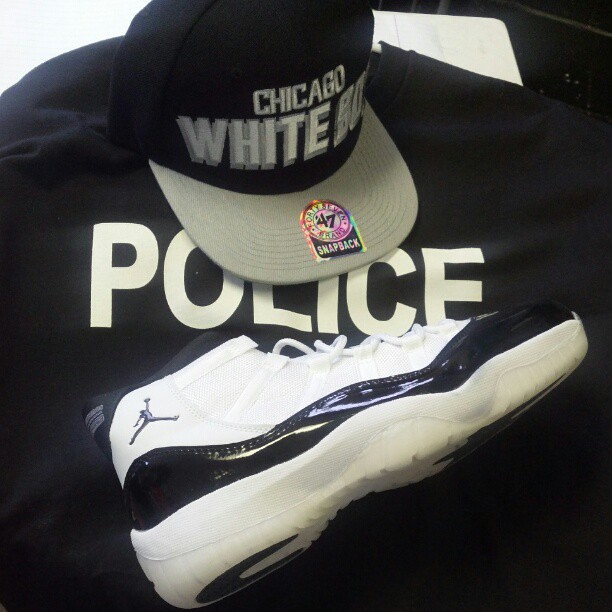This image showcases a carefully arranged outfit taken from above, laid out on what appears to be a bed. At the center, there's a prominent black sweatshirt that boldly displays the word "POLICE" in white, capital letters. Resting atop the sweatshirt is a black and white Air Jordan sneaker, distinguished by its black Air Jordan logo on the back and its white middle section and soles. Positioned towards the top of the image, partially cut off, is a black snapback hat with a gray brim. The hat features a folded-back design and bears the text "Chicago White Sox," though part of this text is obscured due to the angle. A distinctive rainbow sticker with the number 47 is affixed to the brim. The image appears to capture an ensemble that someone might have thoughtfully laid out, either indoors or outdoors.